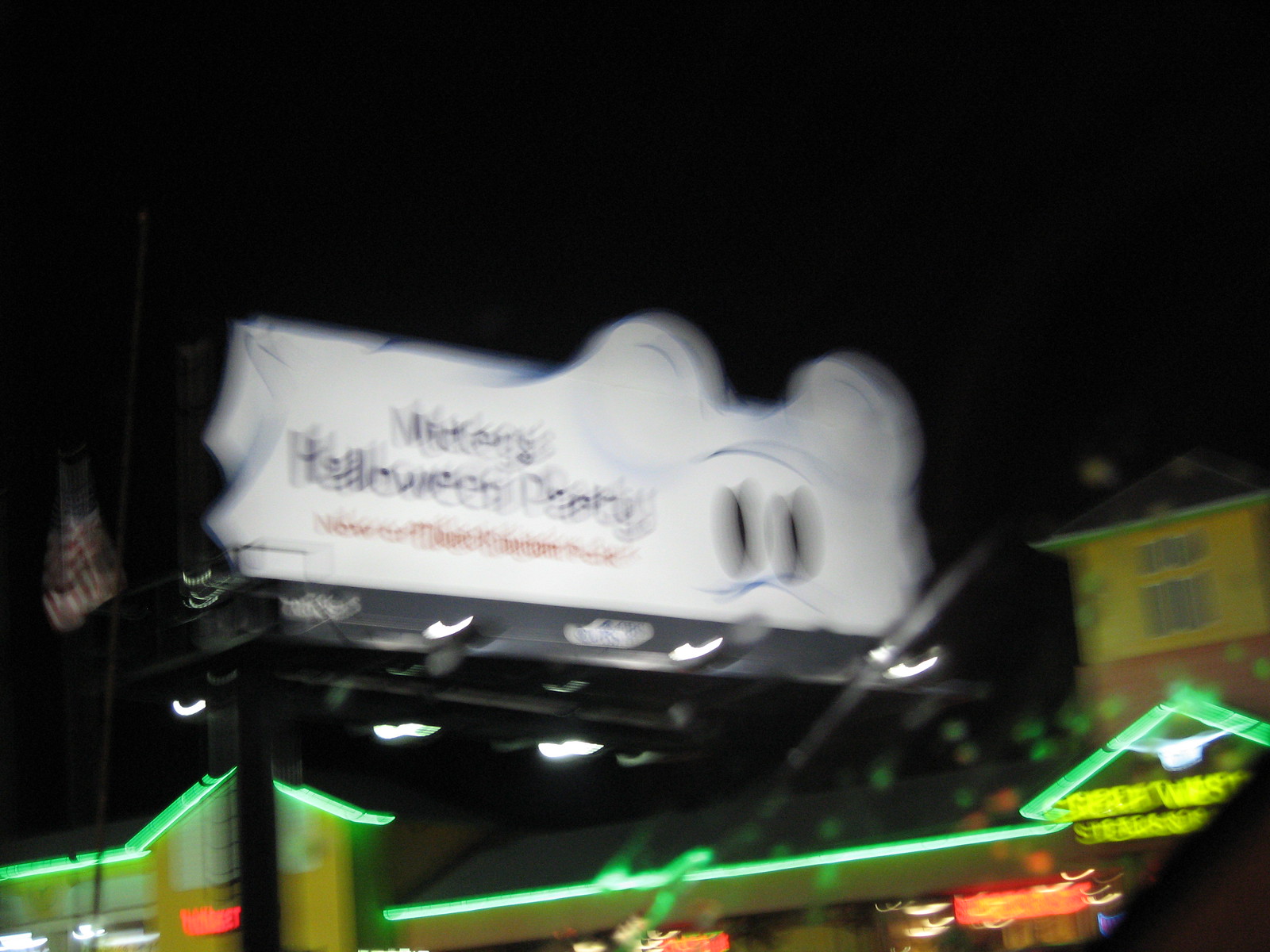An above-ground billboard stands tall on a long, black pole against the night sky. The billboard itself is rectangular but artistically designed to resemble a sheet draped over a rectangular frame. Dominating the right half of the billboard is an image of Mickey Mouse disguised as a ghost, with iconic black eyes peering through the sheet. The left side of the billboard features bold text in black that reads "Mickey's Halloween Party." Below this, in red lettering, it announces "Now at Magic Kingdom," flanked by decorative designs. The billboard is brightly lit, making it a striking sight against the backdrop. In the background, a building that appears to be a hotel with a restaurant attached is visible. The structure is yellow with green neon lights tracing the roofline and red signs glowing in the windows, adding to the night-time ambiance.